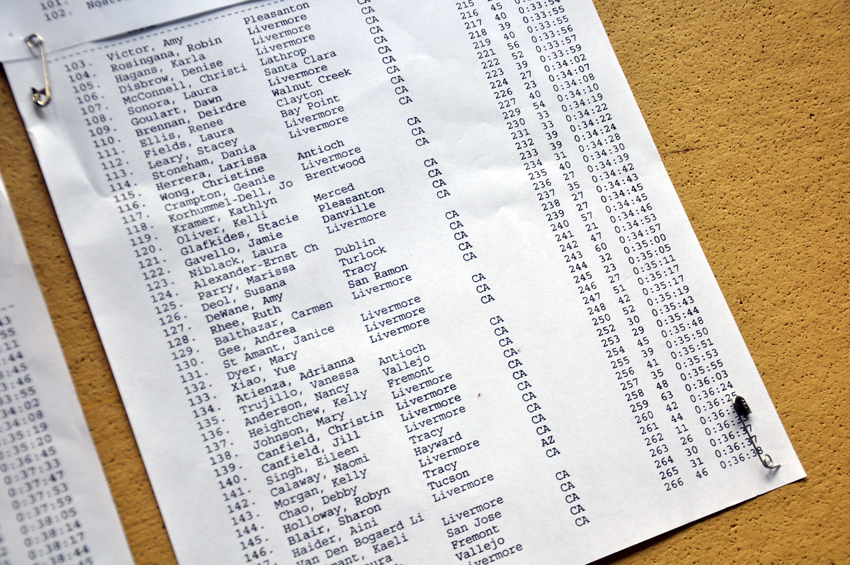The image depicts a detailed call sheet pinned to a corkboard with bobby pins at the top left and top right. The white paper is organized into columns, listing numbered entries starting from 103 and extending beyond 146, featuring locations all within California, such as Pleasanton, Livermore, Lathrop, Santa Clara, Walnut Creek, Clayton, Bay Point, Antioch, Brentwood, Danville, Dublin, Sherlock, Tracy, and San Ramon. Each entry also includes names like Victor, Amy, Rosinga, Robin, Nagan's Carla, Disbrow, and Denise, along with the date and additional numerical data, possibly the duration of the calls. The sheet is part of a publicly displayed notice, providing a clear, black-text-on-white-background presentation of call records.